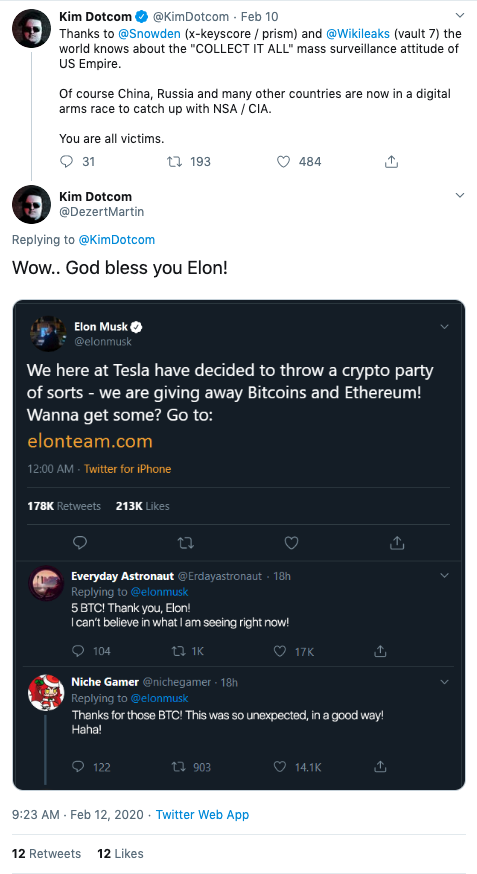### Detailed Descriptive Caption:

The screenshot captures a social media interaction on Twitter, featuring posts by the user kim.com. The conversation unfolds in a series of tweets, highlighting significant topics and user engagement metrics.

**Tweet 1 (February 10th):**
- **User:** kim.com
- **Content:** "Thanks to Snowden and @Wikileaks, the world knows about the all-encompassing mass surveillance attitude of the U.S. Empire. Of course, China, Russia, and many other countries are now in a digital arms race to catch up with the NSA/CIA. You are all victims."
- **Engagement:** 31 comments, 193 votes, and 484 favorites.

**Tweet 2 (Repost of Elon Musk):**
- **User:** kim.com
- **Content:** "Wow... God bless you, Elon!"
- **Context:** This remark refers to a tweet by Elon Musk, which kim.com has reposted.
- **Original Elon Musk Post:** "We here at Tesla have decided to throw a crypto party of sorts. We're giving away Bitcoins and Ethereum. Want to get some? Go to elonteam.com."
- **Visual Details:** Elon Musk's post is displayed in dark mode, contrasted against the light mode of the other tweets.

The image effectively showcases the engagement and interaction between high-profile social media users, focusing on topics related to digital surveillance and cryptocurrency.